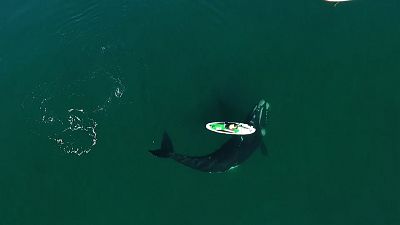An aerial drone captures a breathtaking moment of a paddle boarder, seated on a green-accented, long surfboard, floating serenely in the open dark green ocean. Below the paddle boarder, a majestic whale swims, its body dwarfing the board with a size triple that of the board, characterized by distinctive white spots around its head. The water is clear and smooth, largely undisturbed except for subtle ripples on the left side, possibly a result of the whale's recent movement. The whale's back is arched gracefully, its head pointing towards the top right of the image, creating a uniquely serene and clean visual spectacle amidst the calm, deep green sea.